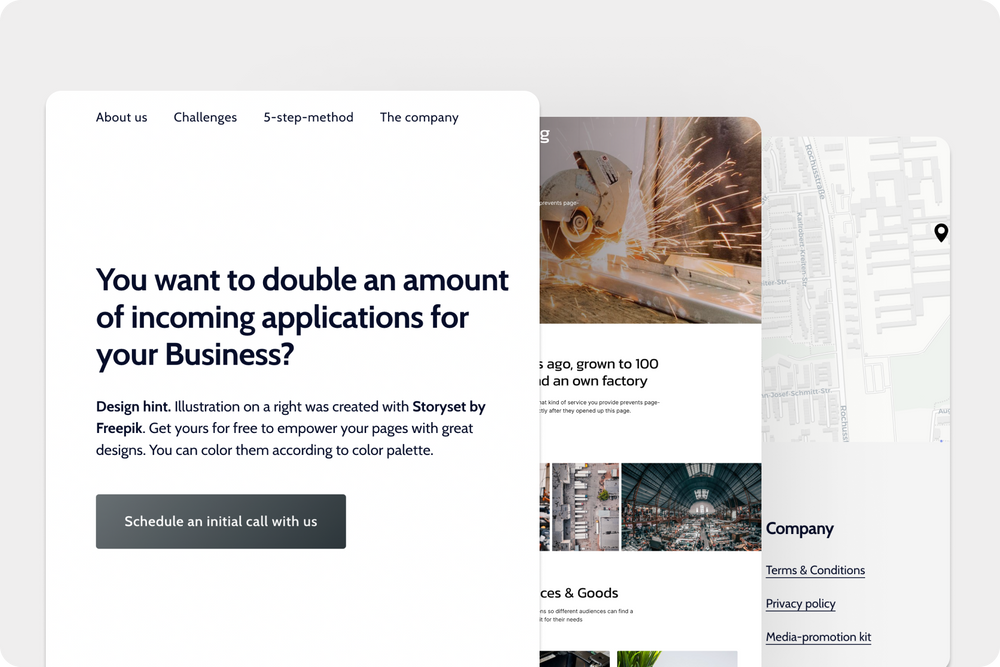This image showcases a pop-up window with three vertically stacked screens, each partially overlapping the one below it. The top screen, positioned toward the left, features a horizontal menu with options labeled "About Us," "Challenges," "S-Step Method," and "Company." Beneath the menu is a large white section containing the text, "Do you want to double the amount of incoming applications for your business?" Additionally, there is a gray button that reads "Schedule an initial call with us."

The middle screen, slightly shifted to the right, displays part of another page. The content visible here hints at a map or geographical representation, extending the informational context.

The bottom screen, aligned further to the right, prominently features the word "Company" on its lower right corner, indicating that this section pertains to company-specific information or branding. The overlapping arrangement and partial visibility of each screen suggest an interactive and layered user interface design.